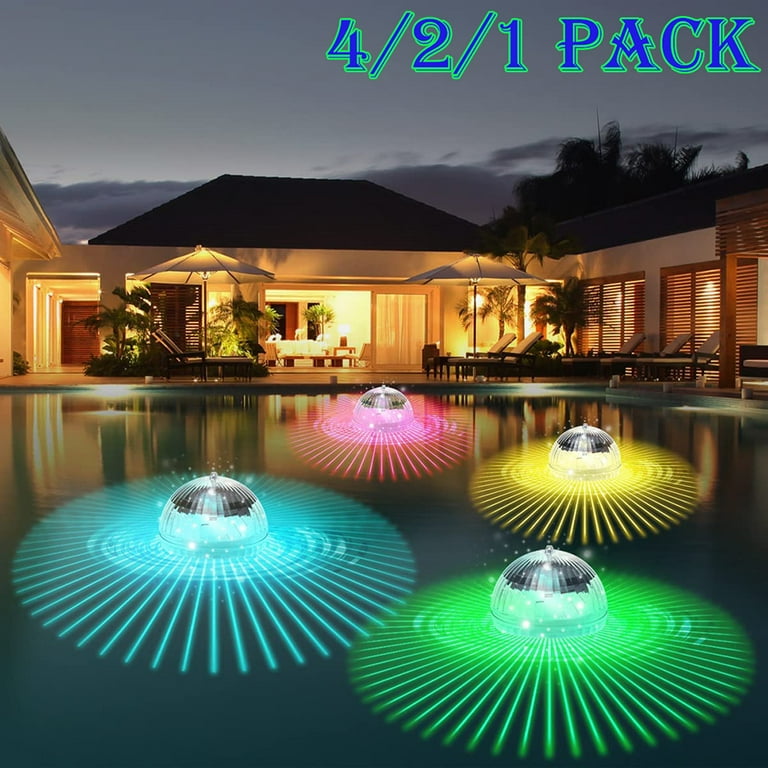The image depicts a nighttime scene of a luxurious tropical resort with a deep blue-green outdoor pool. The resort features a single-story white building with brown wooden doors, framed windows, and wooden posts supporting an overhang, surrounded by palm trees and lush green plants. The sky, transitioning to dusk, is clear with dark red clouds and a grayish hue. The pool area is dotted with lawn chairs and white umbrellas, accentuating the serene ambiance. Floating in the pool are four disco ball floaties emitting vibrant beams of pink, yellow, teal, and green light, creating a dazzling starburst effect. Above the scene, blue text outlined in green reads "4-2-1 PAC," suggesting an advertisement for the disco ball floaties. The setting is both inviting and whimsical, blending tropical tranquility with playful, illuminated decor.